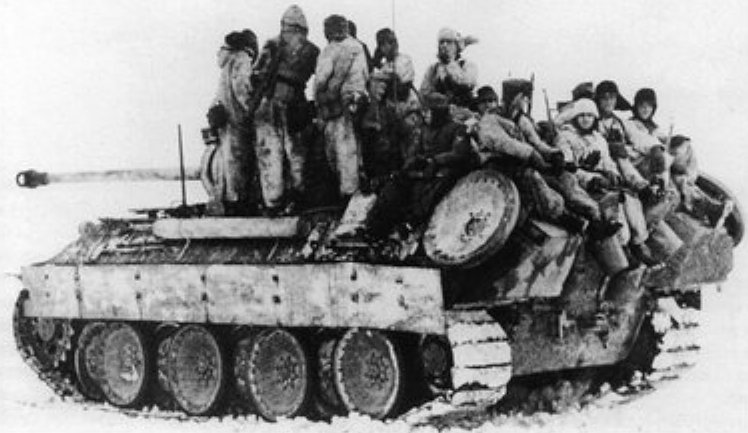This evocative black-and-white photograph appears to capture a moment from World War II, set against a stark, wintry background. Dominating the scene is an old battle tank, its tires and surrounding ground blanketed in snow. Perched atop the tank, a group of individuals huddle closely together, their thick, furry coats and hats indicating the biting cold. Among them, there are both men and women, identifiable through the variance in their attire - some hats and coats appear dark, while others are light. The absence of color emphasizes the contrasts in their clothing and the harsh, snowy environment. The individuals, seemingly soldiers, are not engaged in any overt military activity; instead, one smokes while another gazes directly at the camera, and yet another looks off into the distance, all embodying the stillness of the cold, solemn scene. Although no explicit military uniforms are visible, the presence of the formidable tank supports the assumption of their soldierly roles in this historic, wintry tableau.